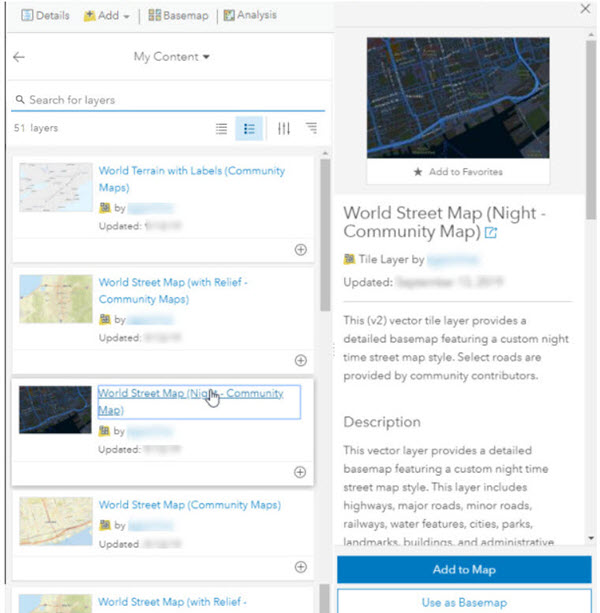The image is divided into two main sections. The left two-thirds of the image has a predominantly white background, with a thin gray border along the top and left side. The top quarter of this segment is light gray, transitioning into white as you move downward.

On the left side, there's a thin gray border along the top. Inside this section, you'll find the word "Details" with an adjacent details icon, and the word "Add" with an adjacent add icon. Below these, several elements appear blurry, including an emblem next to the word "Analysis."

Just beneath, a black arrow pointing left is displayed, followed by the text "My Content" in black, centered on the left side. A search bar appears underneath "My Content." Below the search bar, the text "S1 Layers" is visible, accompanied by four images of maps, each with descriptive information to their right. The names of the maps are displayed in blue text.

On the right-most third of the image, the top features a map. Below the map is a white tab with the text "Add to Favorites" in black, accompanied by a star icon to the left. The map display features blue for streets and green for grass areas.

Underneath the map, in the white section, it reads "World Street Map (Night)" on one line, followed by "Community Map" on the next line with a blue square next to it. Additional informative text is provided on about four lines under this segment, describing the maps or their functionalities. Lower down, a blue tab with "Add to Map" written in white appears, and a white tab below it has the text "Use as Base Map" in blue.